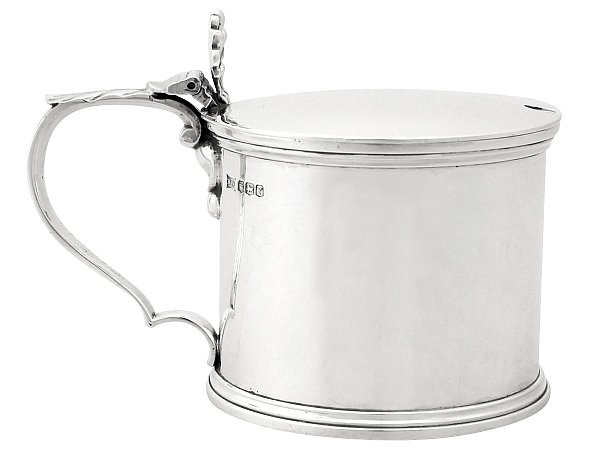This is a detailed photograph of an antique silver cup, resembling a short and stout mug with a wide base crafted from sterling silver. The cup has an attached lid, characterized by a metal handle designed for easy opening with a thumb lever at the top of the handle. The distinctive handle on the left side of the image forms a half upside-down heart shape that further curves into a semi-circle where it attaches to the cup. Below the lid, where the handle is mounted, there are some decorative markings or holes. The entire cup is set against a white background, illuminated by a light source from the left, emphasizing its pure silver metal design.